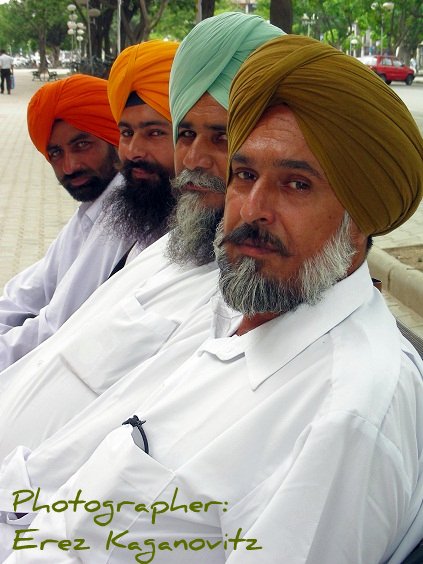This photograph features four elderly men sitting on a bench in a picturesque park. The park's pathways are adorned with light whitish-brown tiles, arranged in six-by-six-inch or four-by-four-inch squares. Greenery and trees form a serene backdrop, and a red truck is visible parked to the upper right, hinting that the park might also accommodate roads.

All four men wear bright white collared shirts and turbans, each of a different color. From left to right, there's an orange turban, a light orange turban, a turquoise turban, and a khaki-brown turban. Each man has a beard of varying lengths and shades: the first man's beard is the shortest and slightly gray, the second's is longer and grayer, the third's is the longest and black, and the fourth's beard is short again.

All men glance directly or slightly turned towards the camera, giving a sense of a moment captured spontaneously. At the bottom of the photograph, text credits the photographer, Eris Kaganovich.